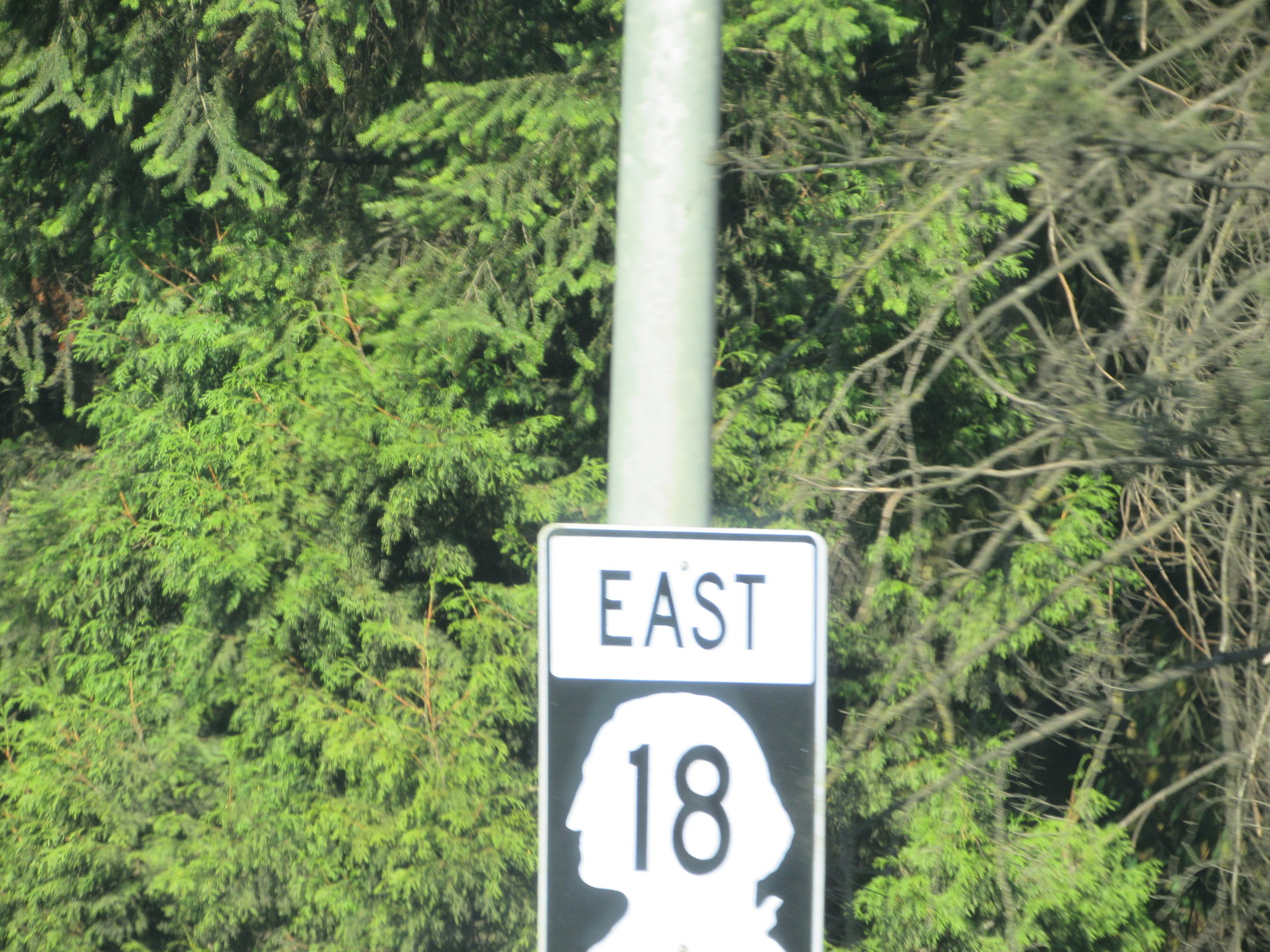The image captures a black and white street sign mounted on a tall silver metal pole positioned centrally in the photo. At the top portion of the sign, "EAST" is displayed in bold black capital letters on a white rectangular background with a narrow black border. Beneath this, there's a prominent silhouette of a man's profile in white, resembling George Washington, facing left. Superimposed on this silhouette is the number "18" in black. Surrounding the sign and pole, the background is filled with various types of trees, including bare and leafy branches, as well as evergreen and pine trees, contributing a mix of gray, brown, and vibrant green hues.